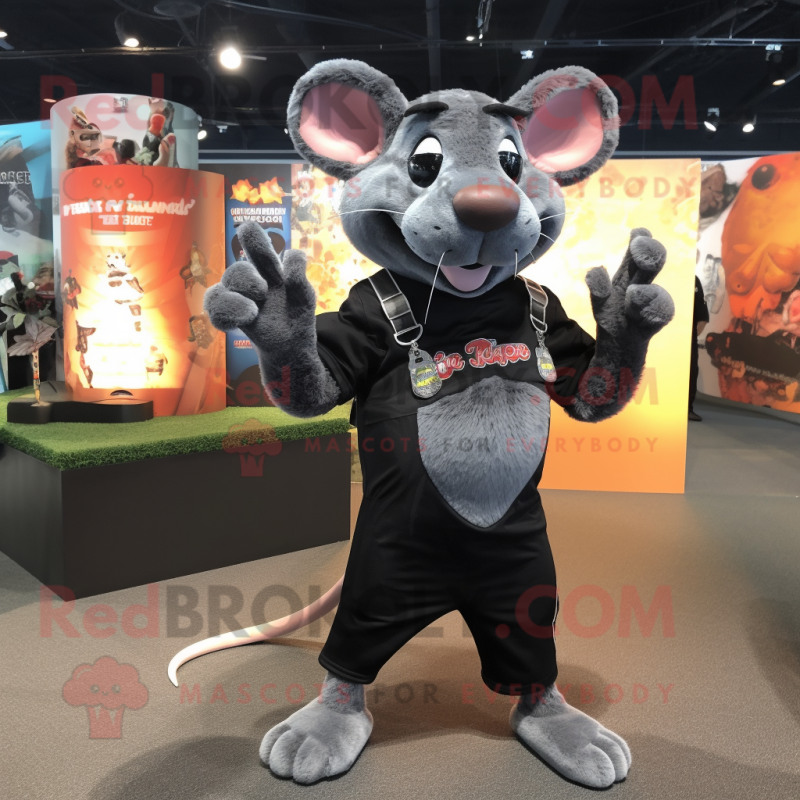In this vividly detailed scene set inside a warehouse-like building, a person dressed in a cheerful, cartoonish mouse mascot costume stands prominently in front of a variety of signs and posters, reminiscent of a museum or event space. The mouse costume features a large gray head with pink ears, expressive egg-shaped eyes that are predominantly black with white tops, a smiling mouth with a small pink tongue, and a brown nose. The mouse is depicted with white whiskers, three on one side and two on the other.

The mascot wears a black short-sleeved shirt, revealing gray fur-covered arms, and black overalls with straps that partially expose a light gray furry belly. The overalls extend down to slightly above the ankles, uncovering furry gray feet. Its pink tail extends out and curves slightly to the left from our viewpoint. The person in the costume has their hands raised and bent at the elbows, with the right hand's pointer finger and thumb up as if making a gesture, while the left hand has fingers bent.

The backdrop includes various large poster boards and placards, with a conspicuous yellow and orange one bearing text that is hard to read due to it being faint and watermarked across the image. The watermark, reading "redbroker.com" with a logo of a red cupcake with black eyeballs, accompanies the slogan "MASCOTS FOR EVERYBODY," hinting at an advertisement for hiring mascot services.

The floor beneath the character is a charcoal gray hard surface, and to the left, there’s a dark brown raised platform with green artificial turf and some indistinct objects on it. Overhead, ceiling lights hang from the warehouse ceiling, casting illumination over the surreal yet inviting scene.